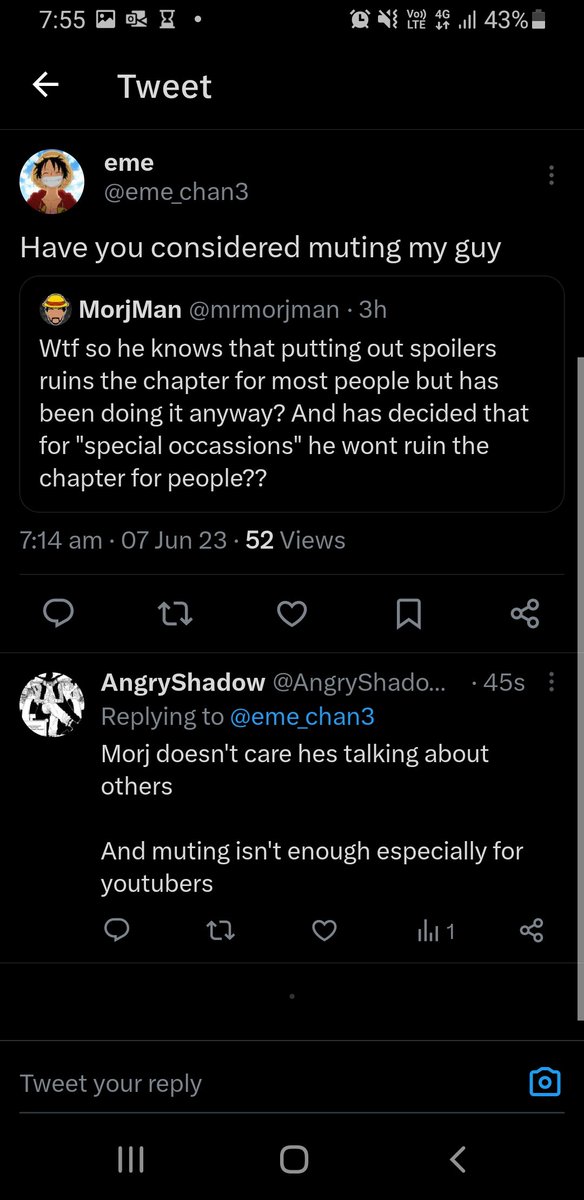This image appears to be a screenshot of a Twitter conversation. In the initial tweet, a user by the handle @Moshman passionately expresses frustration: "WTF, so he knows that putting out spoilers ruins the chapter for most people but has been doing it anyway and has decided that for special occasions, he won't ruin the chapter for people. Mosh doesn't care. He's talking about others and muting isn't enough, especially for YouTubers." In response, a user named Emi (@Emi) replies succinctly, "Have you considered muting, my guy?" This dialogue highlights a heated debate on spoiler etiquette within online communities, particularly emphasizing the challenges faced by content creators and their audiences.